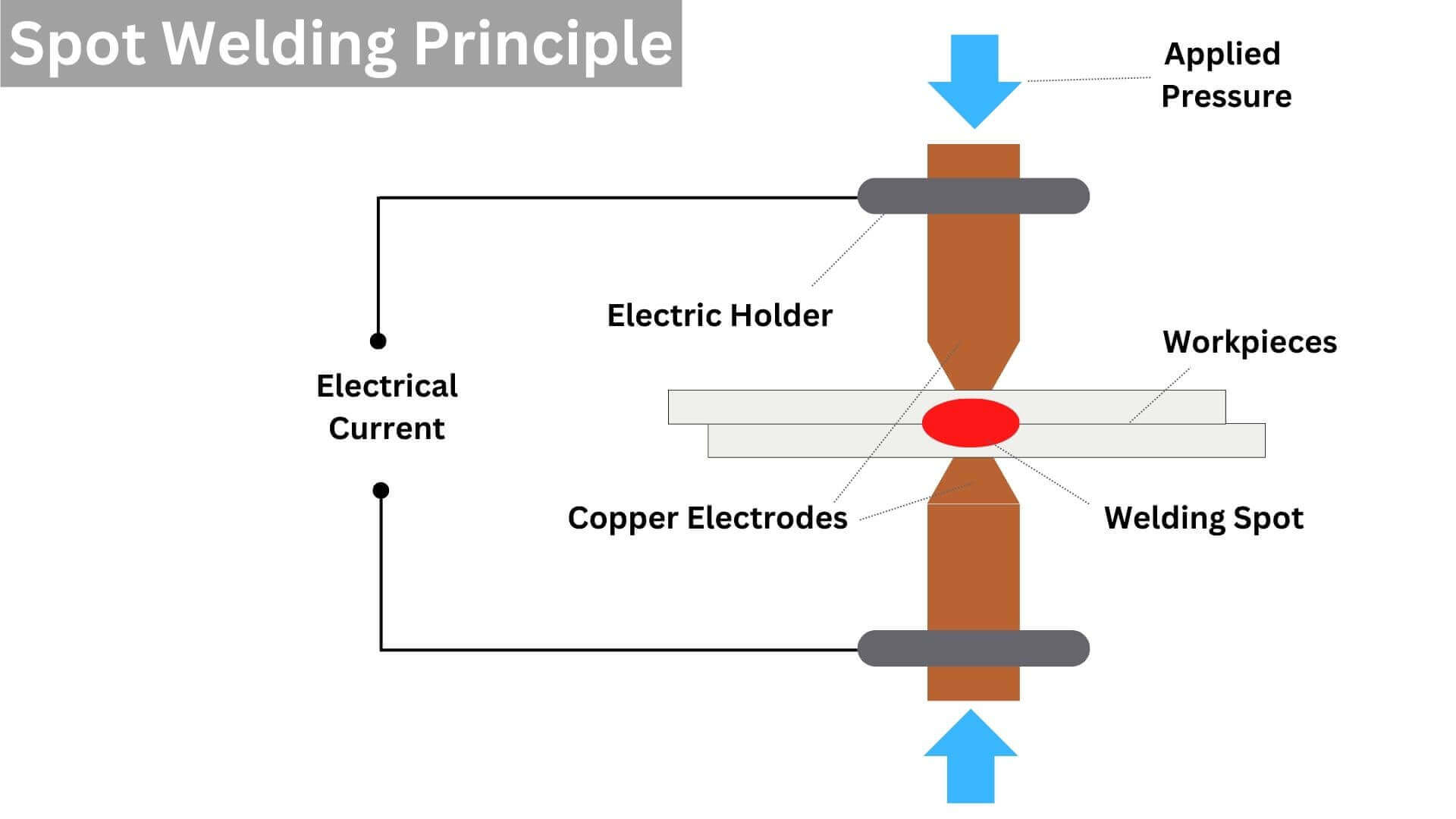This diagram, set against a white background, visually illustrates the spot welding principle. In the upper left corner, a gray bar features the title "Spot Welding Principle" in white text. Central to the image is a detailed depiction of the welding process: two brown copper electrodes, each with a gray electric holder at the top, apply pressure to two metal work pieces. A light blue arrow labeled "Apply Pressure" points downwards from the upper right, emphasizing the force exerted by the electrodes. Between the electrodes, in the central area where they make contact with the work pieces, the term "Welding Spot" is indicated, highlighting the area where the welding occurs. The diagram also annotates the flow of "Electrical Current" necessary for the spot welding process. Each component, from the electrodes to the work pieces, is clearly labeled, making the diagram a comprehensive guide to understanding the mechanics of spot welding.